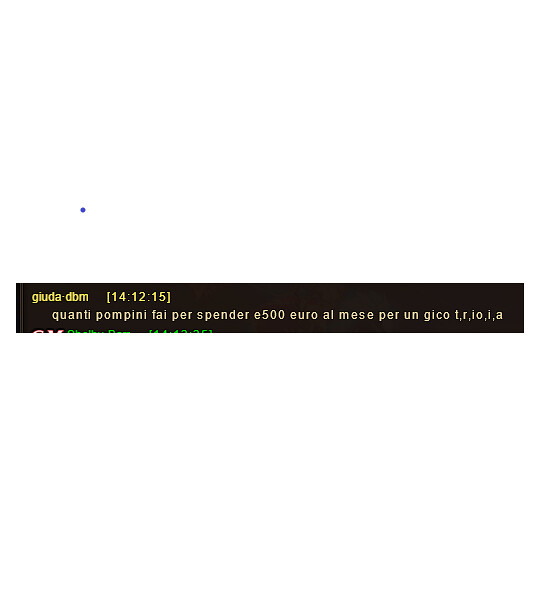The image depicts a small, black rectangular text box, resembling a snippet from a chat room conversation. At the top left corner, it reads "GATA DBM" in yellow font, followed by "(14:12:15)". Below this, an indented line of text in the same yellow font states, "Quanti pompini fi per spender E 500 euro al mese per un gico T, R, IOU, I, A." A blue dot is visible above the rectangle. The text appears to be in a foreign language, possibly Italian, and captures a brief, possibly conversational snippet.